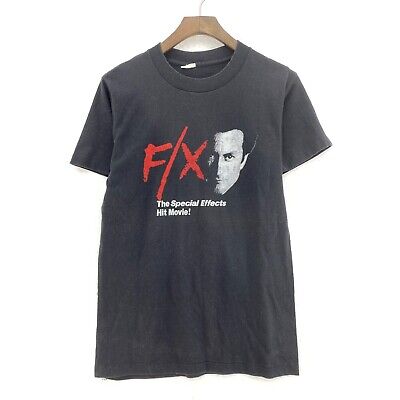This detailed photograph showcases a vintage black cotton t-shirt, short-sleeved with a regular crew neck, hanging on a wooden hanger against a plain white background. The t-shirt features a design inspired by the movie "FX," which is prominently displayed in red text on the chest with the characters "F/X." To the right of this text, there's a striking black-and-white image of the movie's main actor, Bryan Brown, capturing a portion of his face with a severe expression. Below the image, in white text, the slogan reads, "The special effects hit movie!" The black color of the t-shirt appears slightly faded, suggesting it is a secondhand item, and it shows some wrinkles, especially towards the bottom. The overall clean presentation and professional photography hint at the t-shirt being sold, possibly because it is now a rare collectible item. The emphasis on the image and the crisp details provided make it clear that this t-shirt is not only a piece of clothing but also a cherished piece of movie memorabilia.